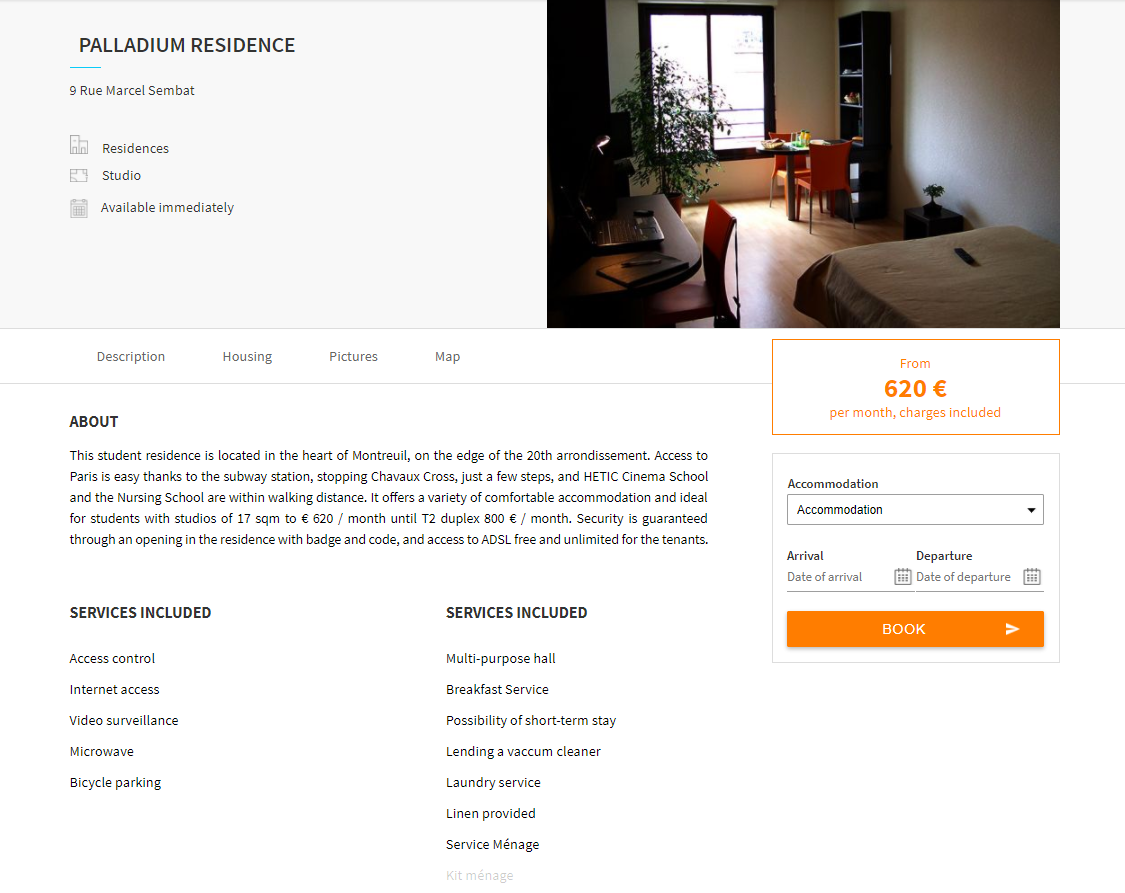**Palladium Residence Advertisement**

In the upper left corner, the image prominently displays the text "Palladium Residence" in bold, all-caps font. On the right side, a photograph showcases a cozy studio room available for rent. The room features a neatly made bed against beige walls, a window on the left wall, and a vibrant green plant adding a touch of nature. A small desk with a laptop sits ready for work, accompanied by a couple of chairs. Adjacent to the bed is a small table topped with drinks and a petite plant, creating a homely ambiance.

The text on the left side of the image provides the address "9 Rue Marcell Simbat" and notes that the residence's studio is available immediately. Beneath this, the categories "Description," "Housing," "Pictures," "Map," and "About" are listed. The description elaborates that the student residence is situated in the heart of Montreal, near the edge of the 20th arrondissement. Access to Paris is convenient via the Cheval Cross subway station, located just steps away. Both HETIC cinema school and the nursing school are within walking distance.

In the bottom left corner, a list of included services is provided: access control, internet access, video surveillance, microwave, and bicycle parking. On the right side, additional included services are mentioned without specifics detailed in the caption.

An orange border in the upper right corner states "from 620," though the currency is unclear. Below this, the text "Accommodation" appears, followed by fields for "Arrival" and "Departure" dates, and an orange "Book" button inviting potential residents to secure their stay.